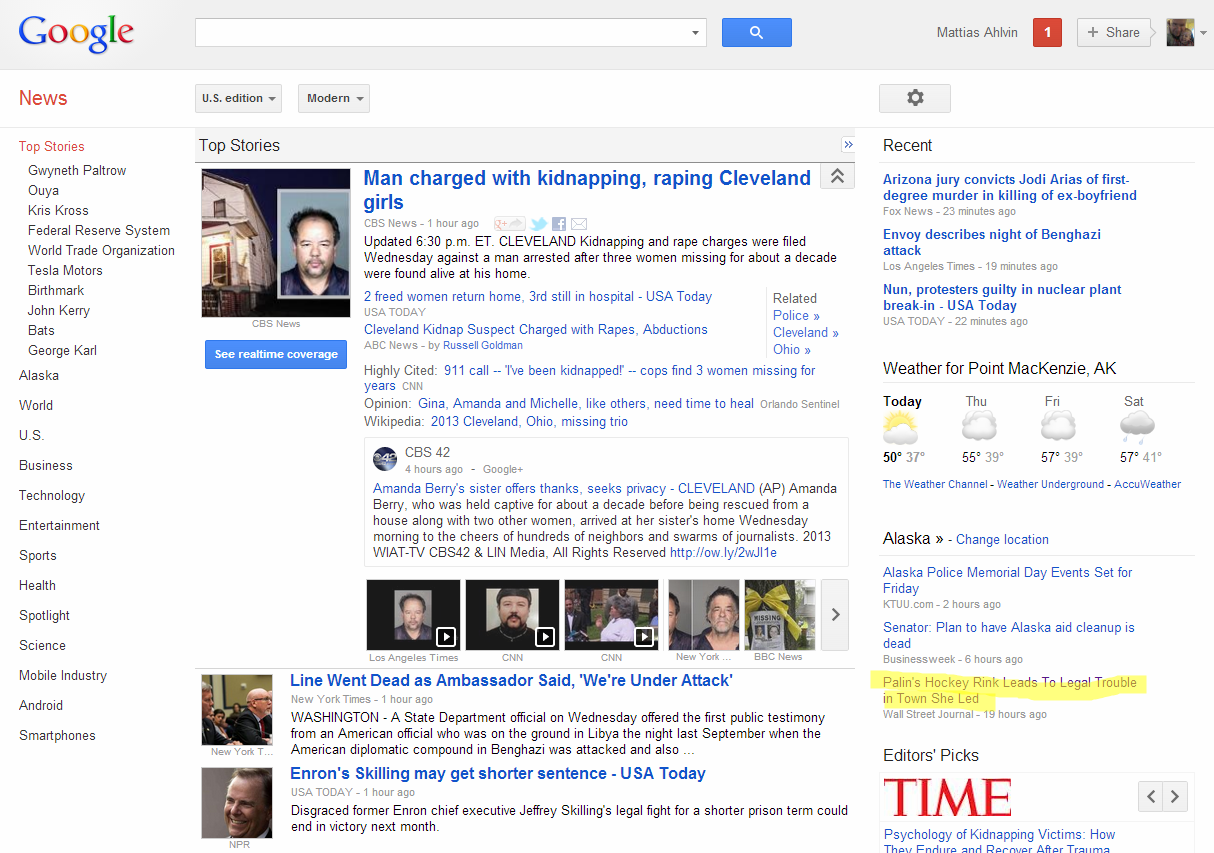This image depicts a classic Google News page with an older design. At the top, a gray bar is visible featuring the Google logo on the left. Adjacent to the logo, there is a search bar. Towards the right, the text "Maltese Alvin" is displayed, followed by a notification icon with the number one, a share icon, and a small profile picture of the account owner.

The main page has a clean, white background. On the far left side, the word "News" is prominently written in red, beneath which lies a menu with various categories. The menu starts with "Top Stories" and includes sections like Gwyneth Paltrow, Crisscross, Federal Reserve System, World Trade Organization, Tesla Motors, Birthmark, John Kerry, BATS, George Karl, followed by other categories such as Alaska, World, US, Business, Technology, Entertainment, Sports, Health, Spotlight, Science, Mobile Industry, Android, and Smartphones.

In the center, the "Top Stories" section is displayed. The first headline reads "Man Charged with Kidnapping, Raping Cleveland Girls," written in blue, accompanied by a small picture to the left showing the man and a home in the background. Below the headline, a few introductory lines are visible along with several hyperlinks. There's also a smaller window below, likely a tweet from the CBS 42 news channel.

The second headline is "Line Went Dead as Ambassador Said 'We're Under Attack'," accompanied by an image featuring several people to the left of the headline. The third headline, "Enron's Skilling May Get Shorter Sentence," is from USA Today and includes an image of a man on the left.

On the right-hand side, there is a settings option at the top, followed by a "Recent" section listing three different news headlines. Below this, there is weather information for Port Mackenzie, AK, displayed for four days. Another section beneath this provides the option to change the location and lists three Alaska-related headlines. At the bottom of the page, there's a small "Editor's Picks" section.